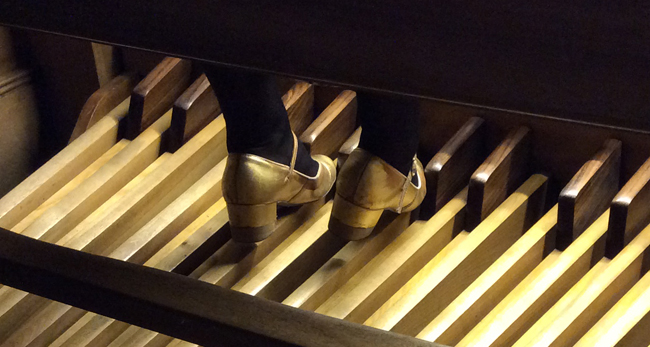The photograph captures a close-up of an organist's feet, adorned in striking golden heeled shoes with brown heels, and wearing black stockings. The feet are delicately positioned on an array of wooden pedals extending the length of the frame, resembling a piano's key layout, but designed for foot operation. The pedals are predominantly of lighter tan wood, interspersed with shorter, darker wooden levers. The detailed arrangement and the way the feet navigate these controls suggest the intricate skill involved in playing the organ. The fragmented, zoomed-in nature of the image focuses exclusively on the feet and the pedalboard, emphasizing the essential role of footwork in the performance.